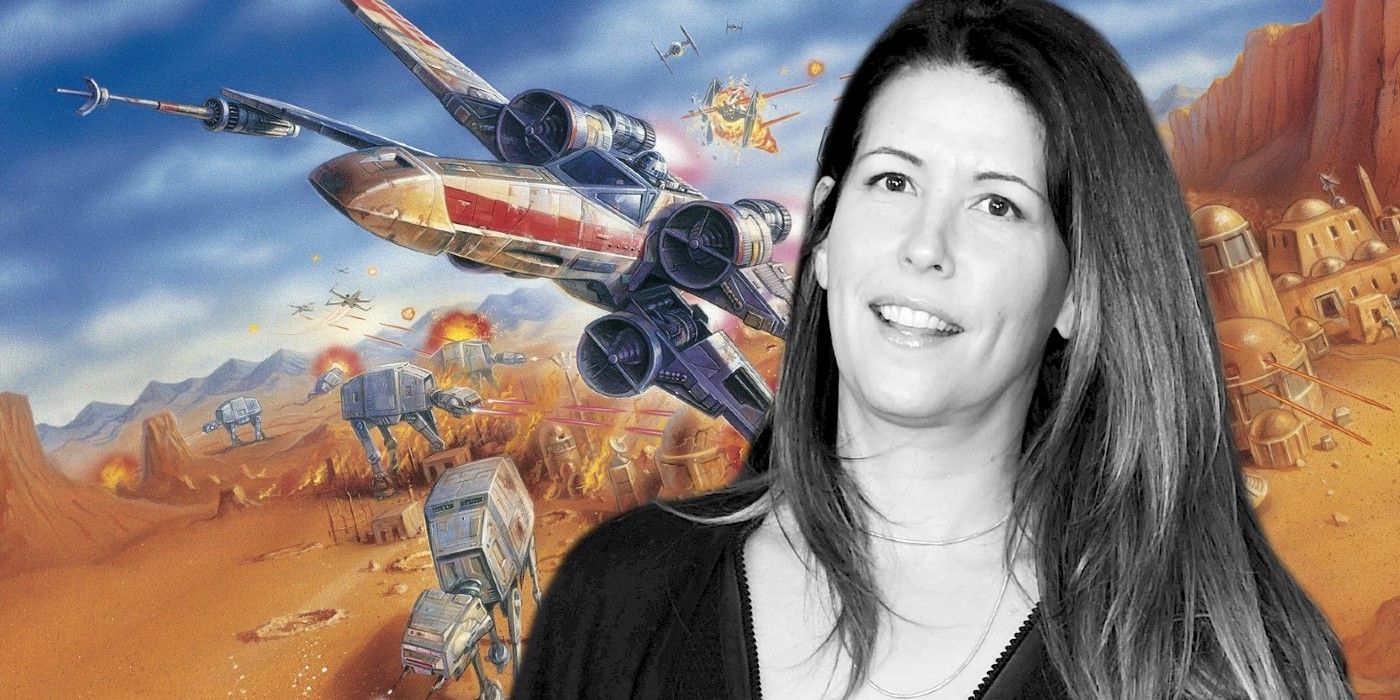In this multi-part image, the background features a dynamic illustration reminiscent of a scene from Star Wars. Dominating the sky, a large gray and red-striped fighter jet charges toward the viewer, accompanied by several smaller crafts. One of these smaller crafts dramatically explodes in mid-air. Set against this aerial backdrop is a desert cityscape, characterized by buildings that resemble sandcastles in their warm, deserty hues. On the ground below, several large, four-legged robotic walkers, bearing a resemblance to metal dogs, traverse the rugged terrain. Scattered craters dot the landscape, adding to the scene's sense of desolation and conflict.

In stark contrast to this vibrant and chaotic illustration, a real-life black-and-white cutout photo of a woman is superimposed in the foreground. The woman has long, straight black hair that cascades past her shoulders. She is dressed in a dark, long-sleeved top with a deep v-neckline that ends just above her chest. Her bright smile reveals her teeth, and her eyes are open, conveying a sense of calm and contentment. This juxtaposition of the real and the fantastical creates a striking and thought-provoking composition.